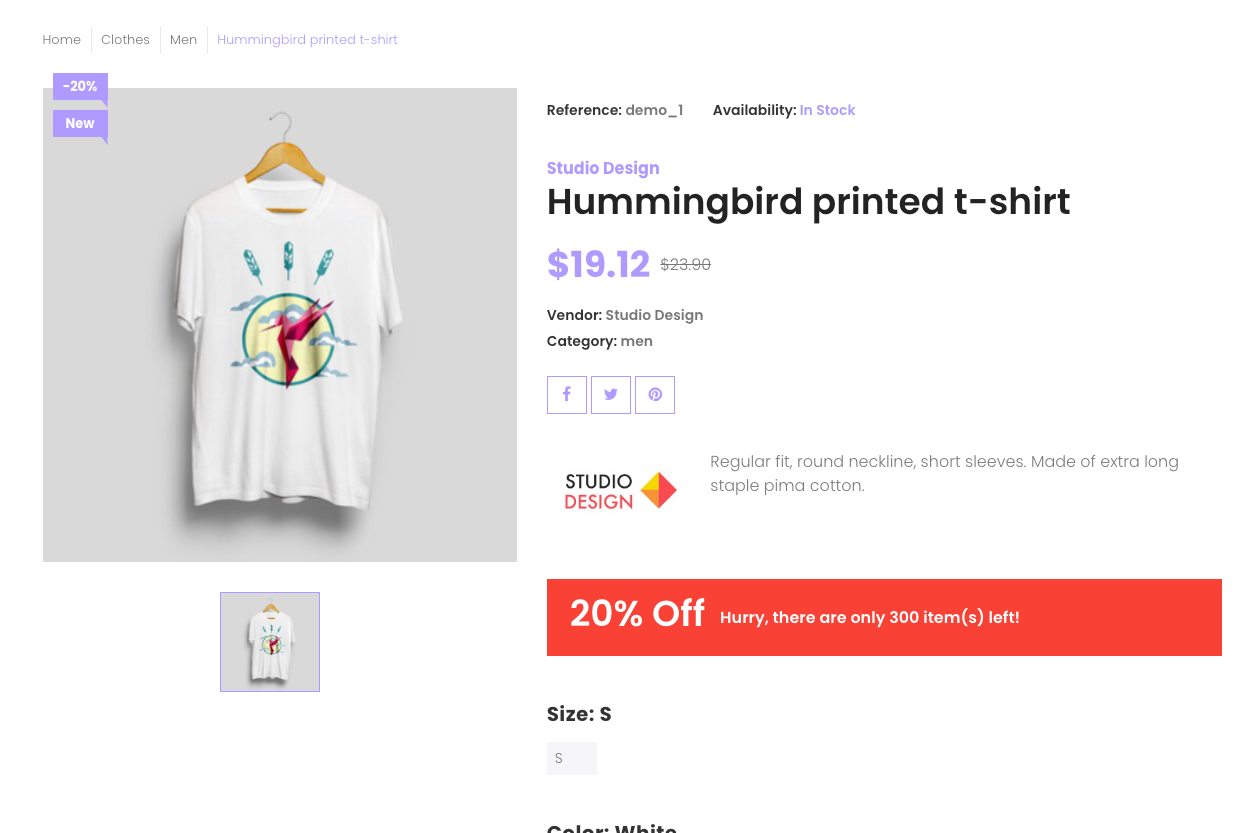The screenshot features a webpage from an online shopping site, specifically highlighting a "Purple Hummingbird Printed T-Shirt" designed for men. The website's navigation bar includes options such as "Home," "Clothes," and "Men." 

The focal point of the page is a large image of the featured t-shirt, which is white with a distinctive design: a yellow circle resembling a sun in the center, overlaid with a pink hummingbird facing left, and three small feathers extending from the top of the circle. Text near the image indicates that the t-shirt is "20% off" and "New," with these labels displayed in purple.

Below the main image, there's a smaller box showing the same picture, suggesting that only one image is available for this product. To the right, product details are listed, including the vendor name "Studio Design," product name "Hummingbird Printed T-Shirt," and the price "$19.12" in purple text.

Additional details note that the t-shirt falls under the "Men" category. Social media sharing options for Facebook, Twitter, and Pinterest are provided, along with the "Studio Design" logo. A prominent orange rectangle beneath this information announces the "20% off" promotion and urges customers to act quickly as only 300 items are left in stock. The size "Small" is currently selected.